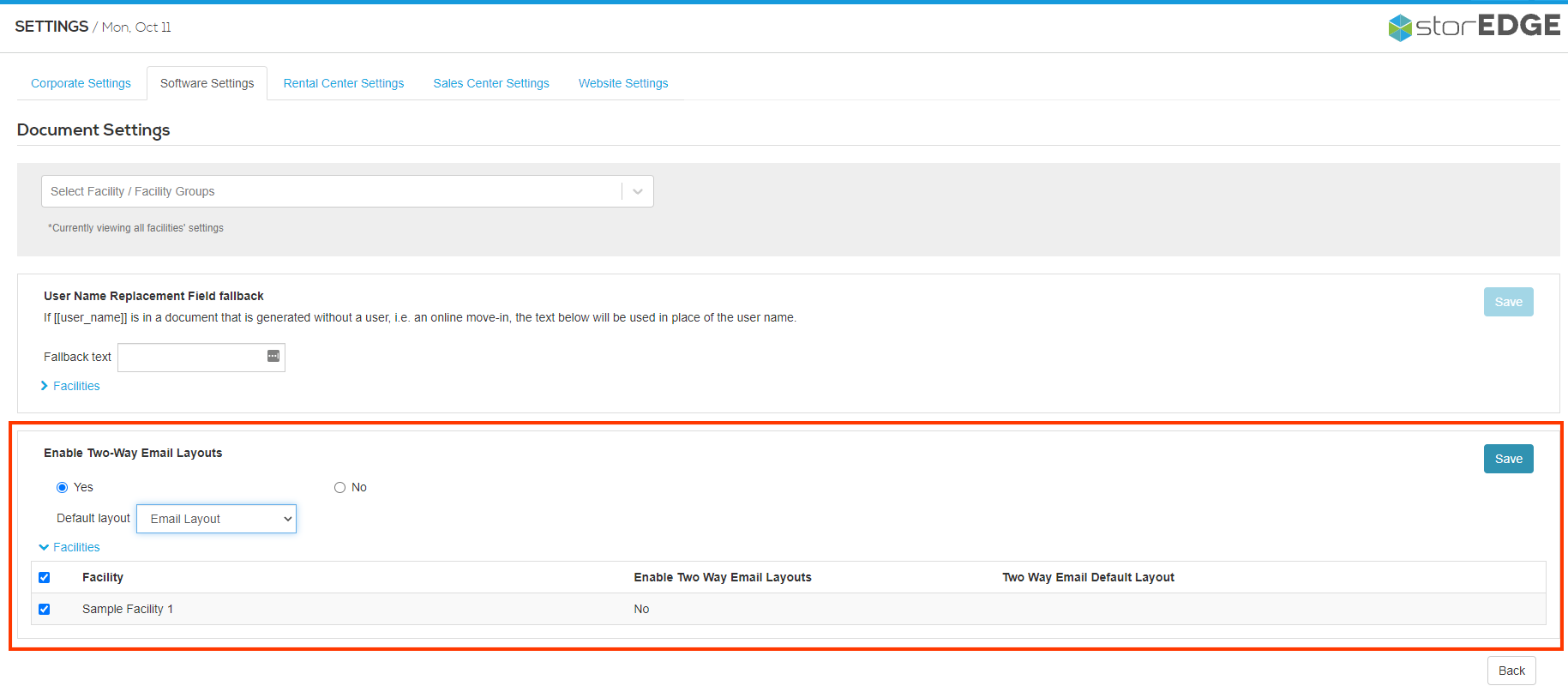The image is a screenshot from a website with a clean, white background. At the top, a thin horizontal blue line spans across the image. In the upper right corner, the text "Settings" is displayed in black, followed by a gray slash, and then the date "Monday, October 11th" in gray. Further to the right, a logo featuring a three-dimensional cube in lime green and blue appears, accompanied by the text "store" in thin lowercase black letters, and "EDGE" in bold uppercase black letters.

Below the top section, there are five navigation tabs aligned horizontally, all in blue except for the second tab from the left, which is highlighted. The tabs are labeled "Corporate Settings," "Software Settings," "Rental Center Settings," "Sales Center Settings," and "Website Settings." The active tab is "Software Settings," and directly below it, a sub-option labeled "Document Settings" is visible.

In the main content area below the tabs, there is a gray box containing a white search field with placeholder text "Select facility, facility groups." Underneath this search box, it displays a statement in gray text: "Currently viewing all facilities settings."